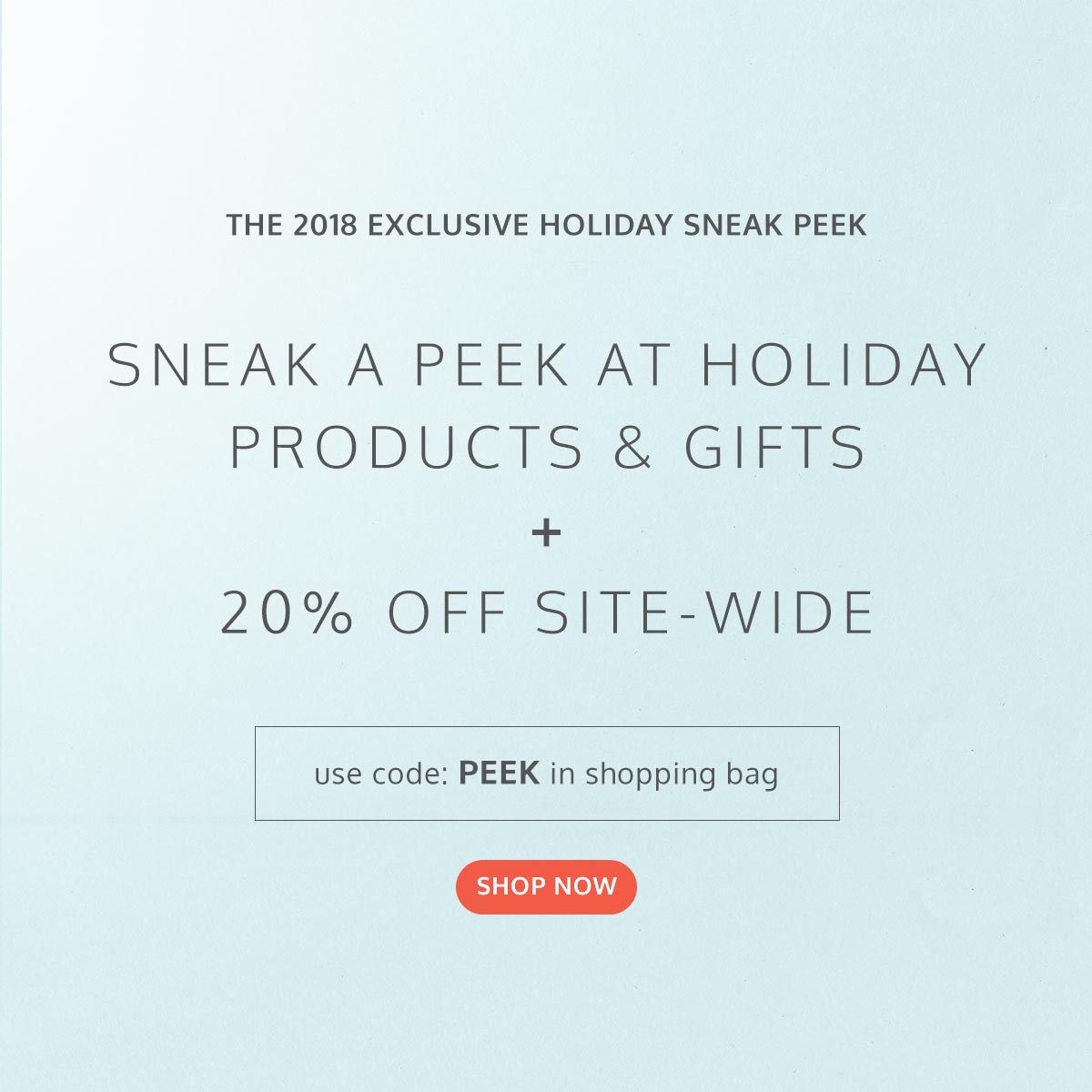The image is a vertically-oriented rectangle slightly taller than it is wide, with a light blue background that fades to almost white in the upper left corner. Centered text dominates the image, starting with "The 2018 Exclusive Holiday Sneak Peek" in black letters at the top. Below this, in larger black letters, is the phrase "Sneak a Peek at Holiday Products and Gifts Plus 20% Off Sitewide."

Further down, a rectangular border encloses instructions to "Use code: PEEK in shopping bag." Beneath this, there's an orange, oval-shaped button with the text "Shop Now" in white letters, suggesting it is clickable. No specific website is mentioned in the image.